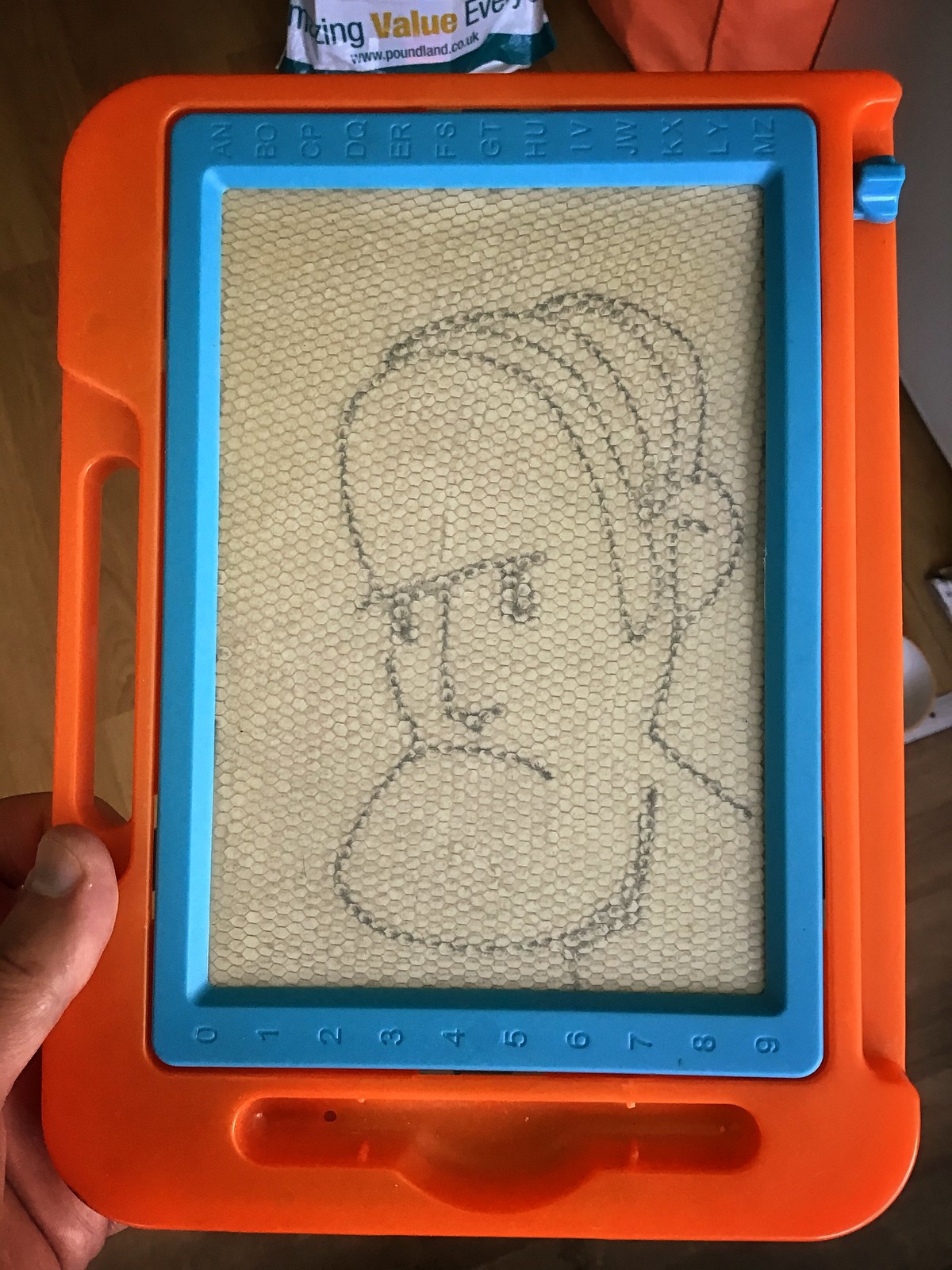The color photograph captures a children's toy reminiscent of an Etch-A-Sketch from the 90s or early 2000s. The toy features a magnetic drawing pad with an orange plastic outer frame and a blue inner frame surrounding a grid-like, light grey screen composed of small hexagons, resembling a honeycomb pattern. The screen showcases a detailed line drawing of a grumpy man with a pronounced chin, combed-back hair on the top of his head, and no fringe. The image looks like a pencil sketch on paper. A blue lever located in a vertical recess at the top right of the orange frame is designed to clear the screen by sliding up and down. A visible left hand, with a thumb grasping the toy, suggests someone is holding it against what appears to be a room floor background.